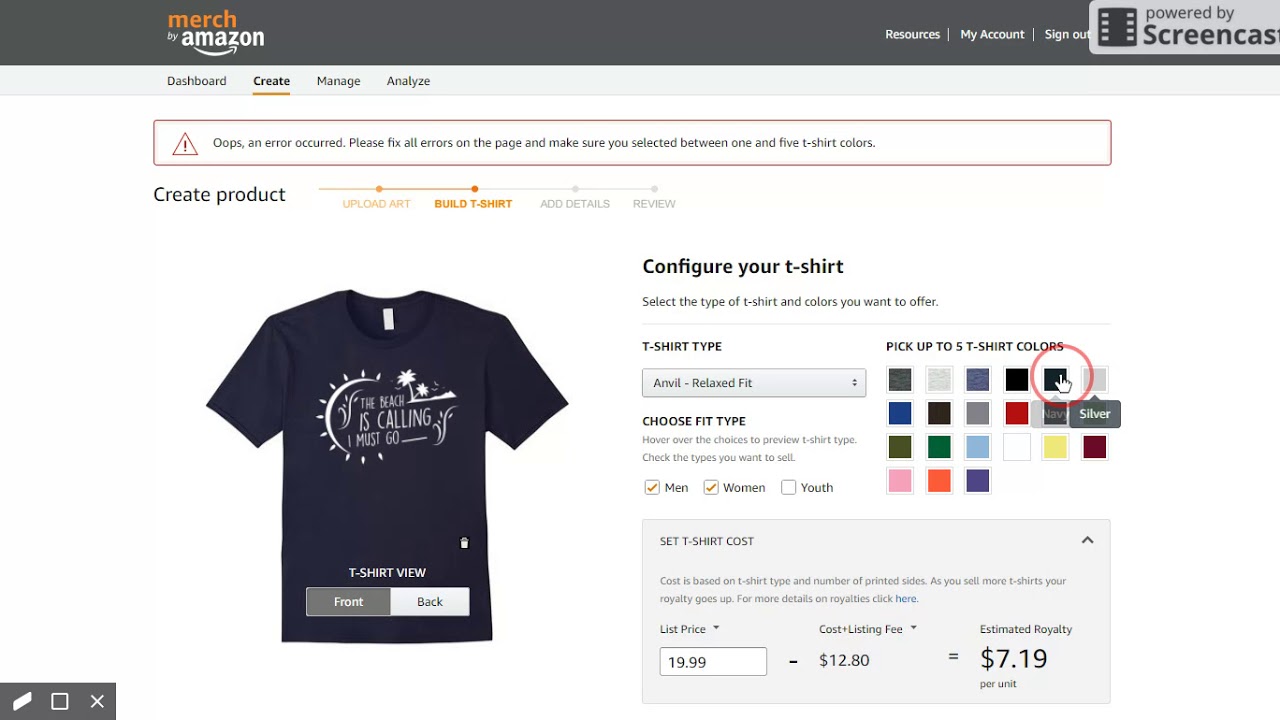This image is a cropped screenshot of the Merch by Amazon store interface. In the top left corner, the label "Merch by Amazon" is clearly visible. On the far right at the top, there is a partially cropped grey box indicating "Powered by Screencast," with the "T" and the right side of the box cut off. Immediately below this header is a thin grey bar spanning the width of the image.

Underneath the header, the sidebar on the left displays four categories: Dashboard, Create, Manage, and Analyze, with "Create" currently selected. The main body of the webpage features a white background. At the top of this section, a red banner alerts the user with the message: "Oops! An error occurred. Please fix all errors on the page and make sure you selected between 1 and 5 t-shirt colors." This indicates that an error occurred because the user did not select the required number of t-shirt colors when attempting to create a product.

On the far right of the page, there is a color selection panel. A hand icon is seen hovering over the black color option, and a red circle has been edited onto the screenshot to highlight this area. This edit is meant to guide the user on where to click to select t-shirt colors.